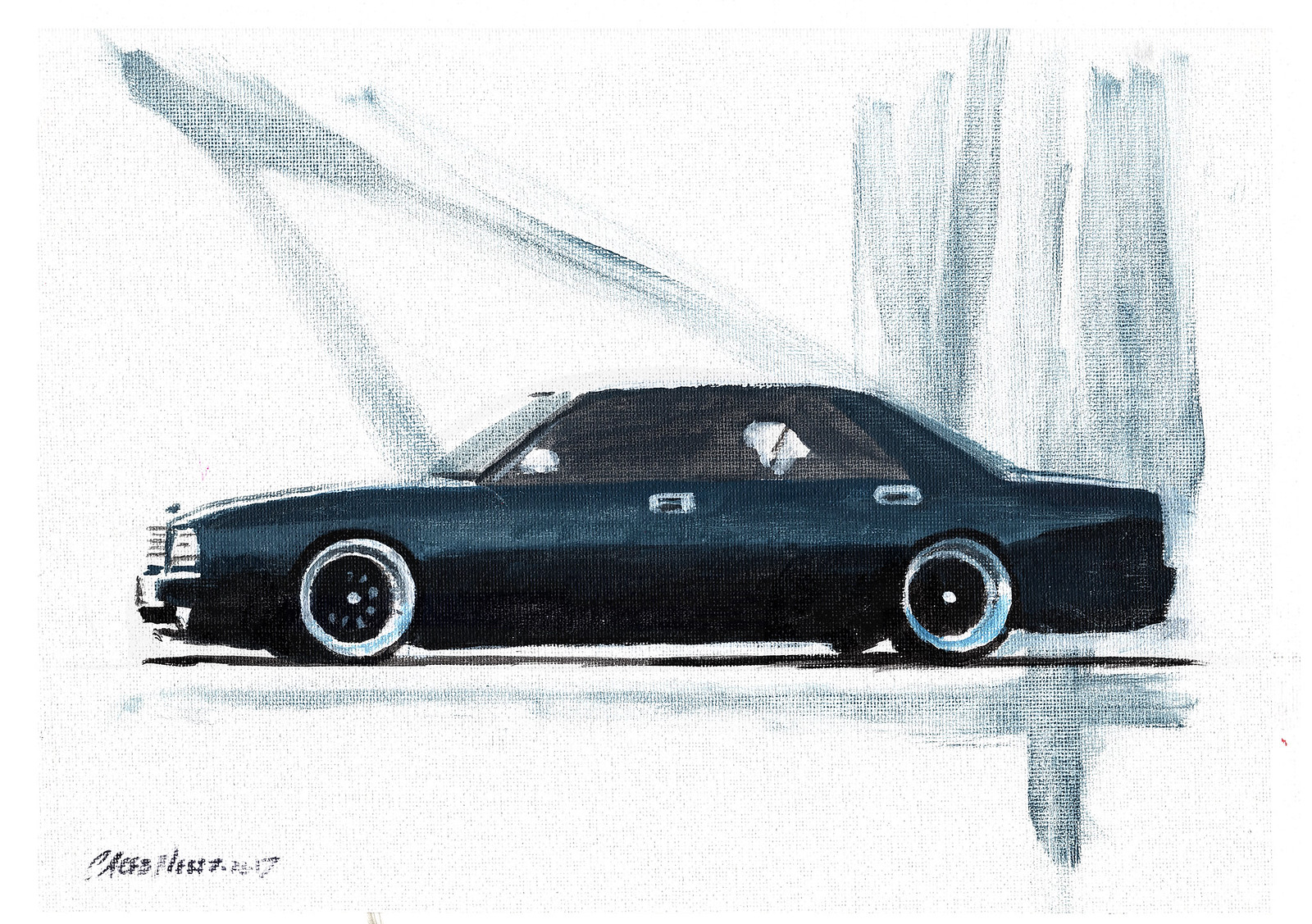This painting, set on a slightly off-white canvas, features a detailed depiction of a luxury Lexus four-door sedan in charcoal black. The car's sleek, modern design is highlighted by its black-tinted windows and distinctive thin tires with large, round chrome rims that have black centers. The vehicle is angled to display its right side while slightly revealing the front, offering a glimpse of the front grille, the left headlight, and a decal on the hood. The background and the area beneath the car are accentuated with subtle neon navy blue shading, adding depth and contrast to the composition. The artist's signature is elegantly placed at the bottom left of the canvas, completing this visually striking automotive portrait.